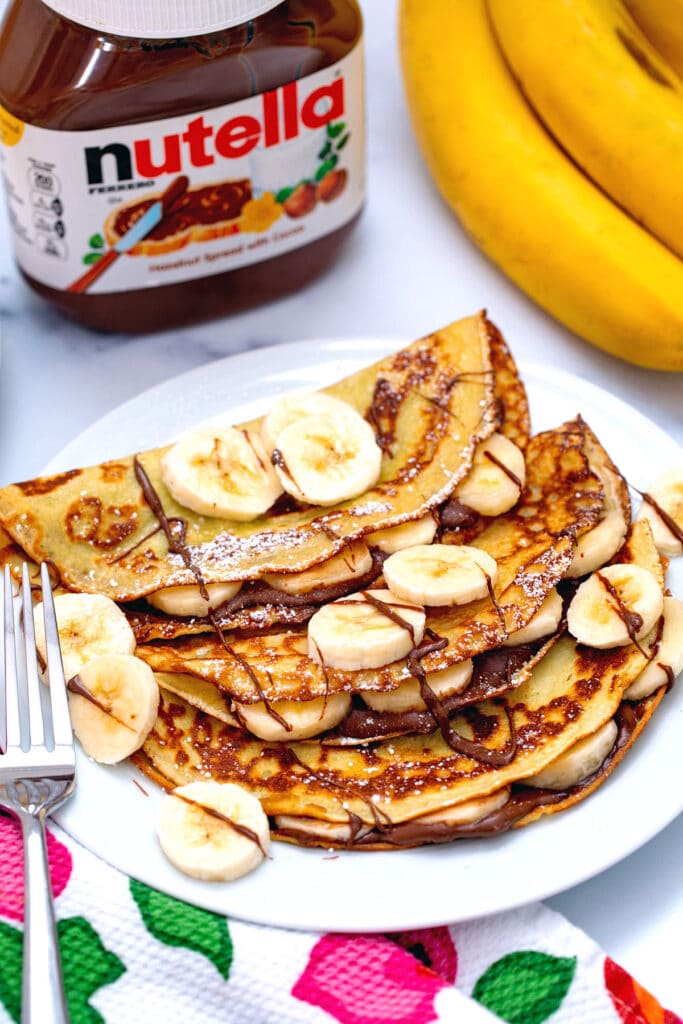This vertical rectangular image showcases a delectable breakfast, likely presented as part of an advertisement for Nutella. At the center of the image, a white plate holds three thin, crepe-like pancakes that are neatly folded over. These golden-brown crepes are filled with sliced bananas and Nutella, with some Nutella visibly drizzled atop them. Additional banana slices are used to garnish the plate, adding to the overall presentation. A transparent plastic jar of Nutella with a white lid and its distinctive brand label, featuring "Nutella" in black and red letters, sits in the upper left corner. The Nutella jar label also includes an image of a toast spread with the chocolate hazelnut spread using a knife. To the upper right, a bunch of ripe yellow bananas, one with a small dark spot, emphasizes the freshness of the fruit. An elegant silver fork is placed to the left of the plate, atop a white napkin adorned with a strawberry and green leaf pattern. The background appears to be a white countertop with gray marbling, which enhances the clean, appetizing presentation of this breakfast setting.